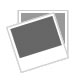The image depicts a close-up of a vintage war medal clasp, positioned on a folded red, white, and blue ribbon. The ribbon, which appears to be made of a polyester cotton blend, features two lines each of red, white, and blue running vertically from top to bottom, and is visibly worn, with brownish blood stains on the left side. The clasp itself is an antique pewter color and takes on a star-shaped design emanating from a central medallion. This medallion features a keyhole cutout and is bordered by four extensions resembling triangles, each engraved with worn letters: an 'M' on the right, an 'M' on the bottom, a 'T' on the left, and an indeterminate letter at the top. The ribbon appears doubled over with creases at the bottom, highlighting its aged and possibly military origin.